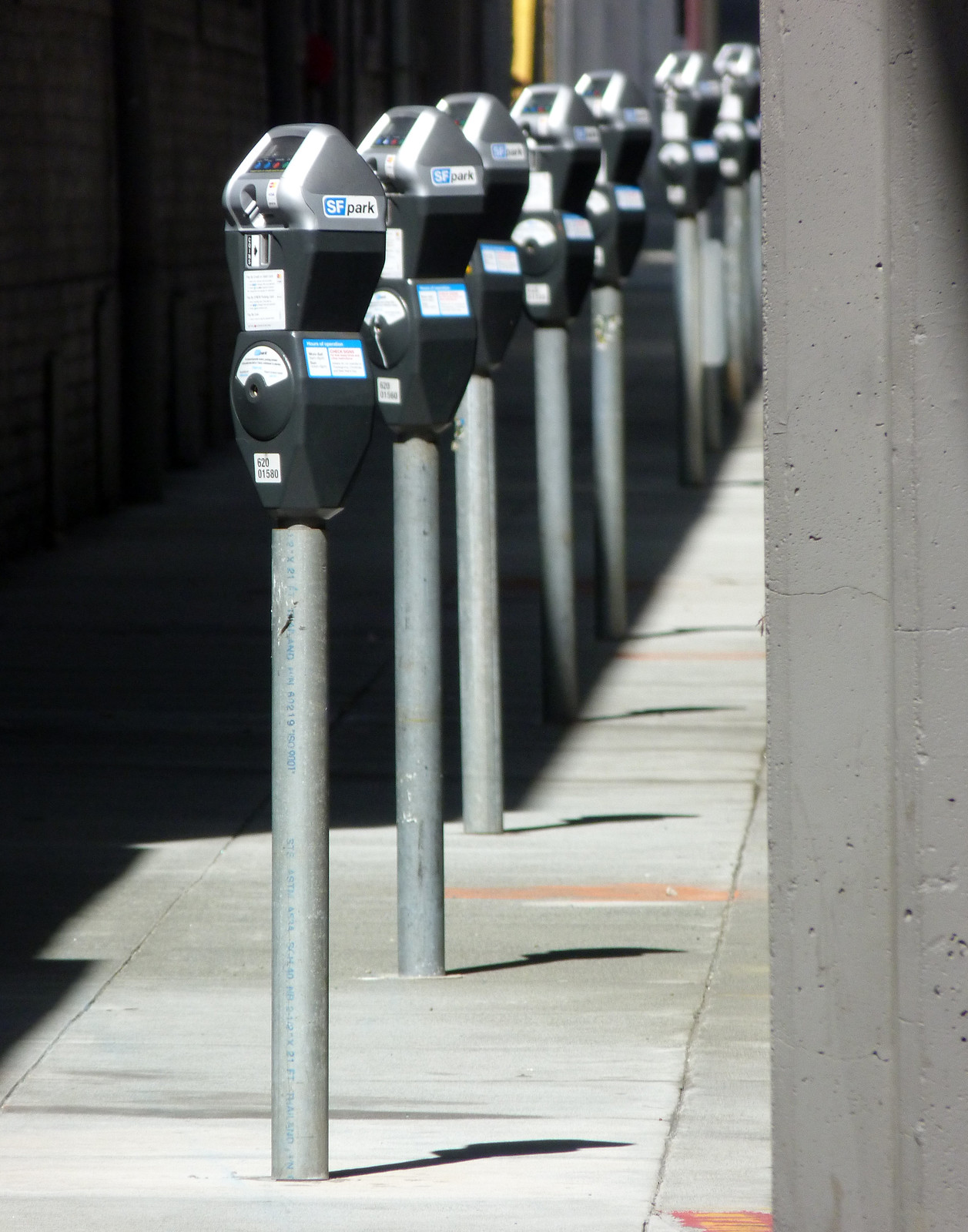This photograph captures a row of parking meters lined up along a concrete-tiled sidewalk. The parking meters, each mounted on a steel post, feature a black housing with a silver top that holds the meter mechanism. The silver top displays "SF Park" on its side. The perspective of the image shows the closest parking meter in the bottom middle-left quadrant, extending down the row to the last, smaller meter in the upper right middle quadrant, creating a sense of depth. On the right-hand side, a cement post of taupe color runs vertically through the scene, while shadows cast along the left side reveal the brick walls of adjacent buildings.